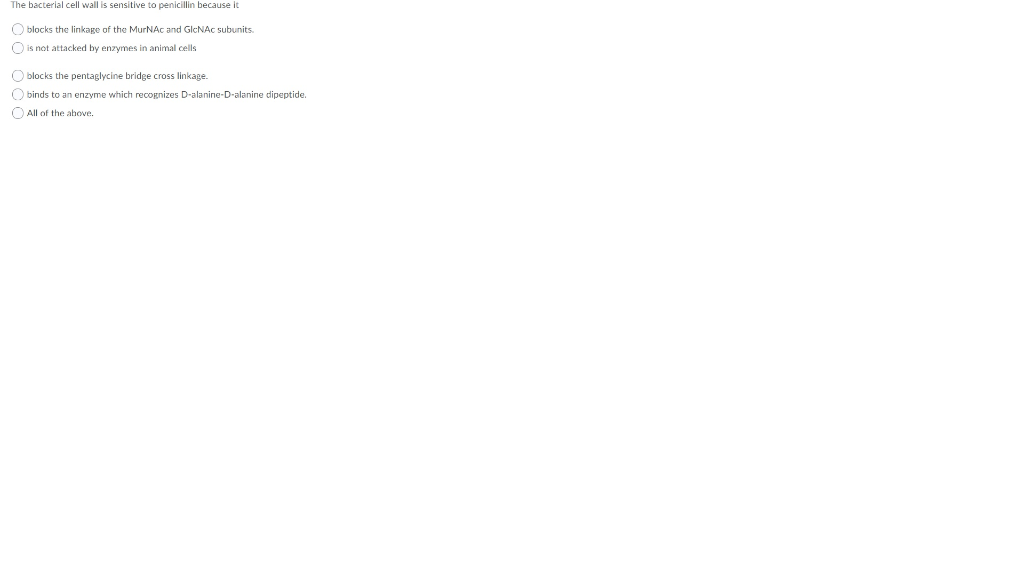Image Description: 

The image features a multiple-choice question examining the sensitivity of bacterial cell walls to penicillin. The question is: "The bacterial cell wall is sensitive to penicillin because it:" followed by five answer options. The options are as follows:

1. Blocks the linkage of the MurNAc and GlcNAc subunits.
2. Is not attacked by enzymes in animal cells.
3. Blocks the pentaglycine bridge cross-linkage.
4. Binds to an enzyme that recognizes D-alanine, D-alanine dipeptide.
5. All of the above.

Currently, none of the answer choices have been selected by the user. The format allows for only one answer to be chosen by selecting the corresponding circle next to the desired option. The image uses a simple black text on a white background, without any additional graphics or imagery. The question is scientific, specifically focusing on biology and cellular mechanisms.